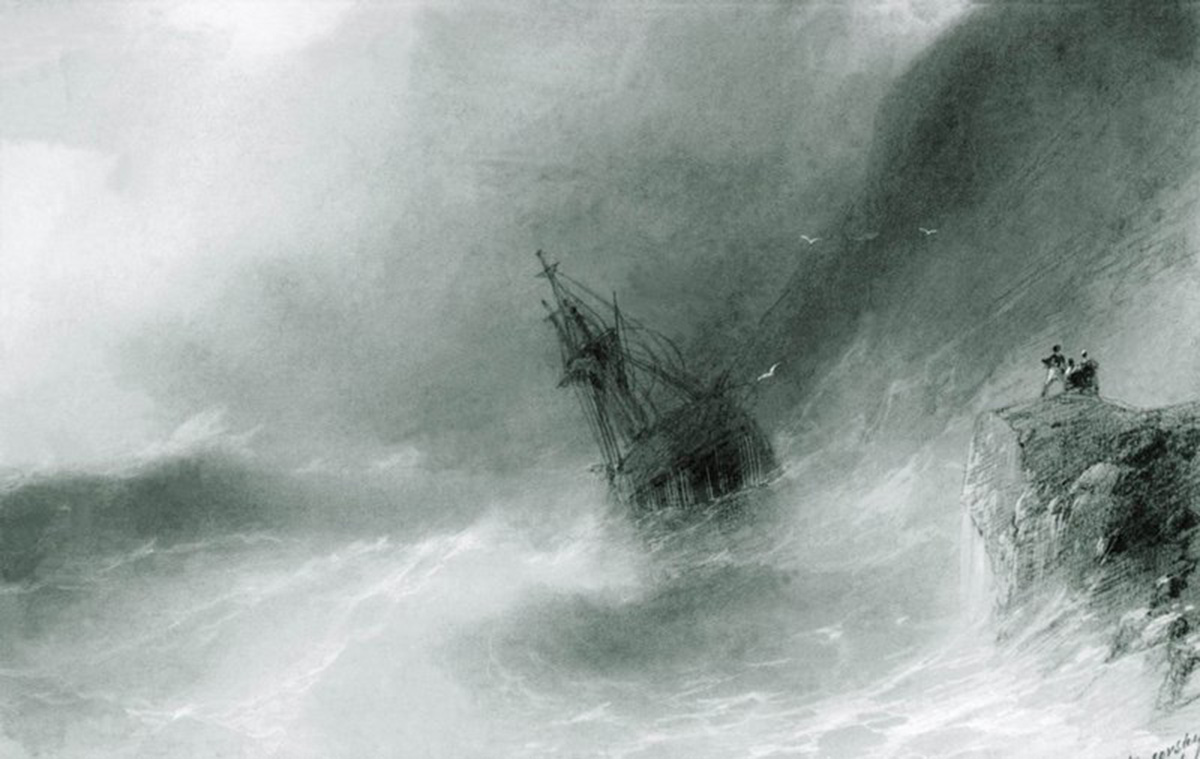In this haunting black and white painting, almost resembling a detailed sketch, an old sailboat battles a violent storm at sea. Dominating the composition, the vessel, leaning precariously to the left, appears as a ghost ship, dark and seemingly deserted. To the storm-battered right, towering waves loom ominously, threatening to engulf the vessel at any moment. White seagulls, numbering four, are scattered, riding the wind on this tempestuous right side. On the rugged cliff to the far right, three figures stand as silent witnesses to the boat’s struggle, their eyes fixed on the dramatic scene unfolding before them. The upper left corner of the artwork is slightly brighter, hinting at sunlight piercing through the chaotic, white-clouded sky, casting a stark contrast. This intricate monochromatic depiction captures the sheer ferocity of nature's wrath, presenting a vivid, turbulent tableau of survival against immense odds.